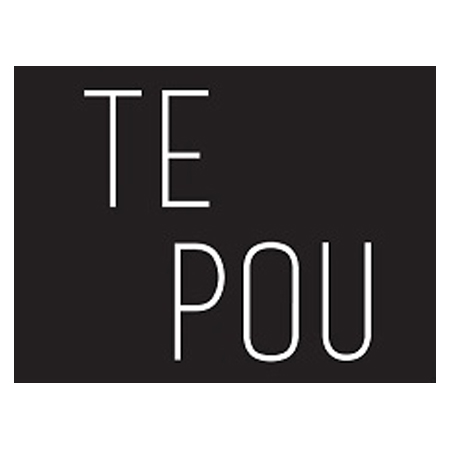The image features a simple, minimalist design with a solid black square background. Positioned within this black square are two words printed in large, white, capitalized letters. The top word, "TE," is slightly offset to the left of the image, while the second word, "POU," is positioned towards the right, directly below the "E" in "TE." This alignment creates empty spaces in the bottom left and top right corners of the image. The stark contrast between the white text and the black background enhances the visual impact of the design.